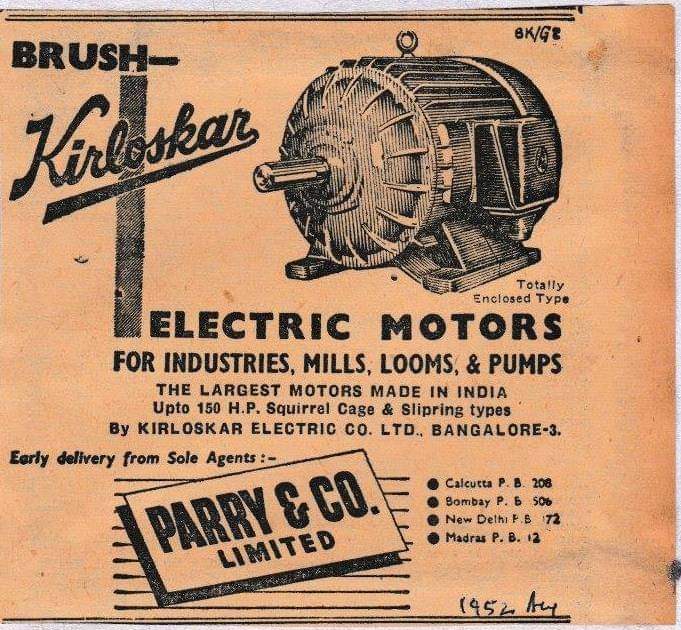This detailed caption weaves together elements from all three original captions:

This monochrome old advertisement, dating back to 1952, appears on aged, yellowed paper with water stains, adding to its vintage charm. Displayed centrally is a detailed illustration of an electric motor, identified by a cylindrical turbine structure with a central shaft and two supporting legs. This motor is promoted by Brush KIRLOSKAR, a name showcased in elegant cursive on the upper left of the ad. Situated beneath the motor image, the ad describes the product as electric motors for various industrial applications including industries, mills, looms, and pumps. It also emphasizes that these are the largest motors made in India, available in up to 150 horsepower, both in squirrel cage and slip ring types. The manufacturer is Brush KIRLOSKAR Electric Co. LTE, and the address indicates Bangalore as its location. Additionally, the ad notes "early delivery from Sole Agents," featuring the logo and name of Parry & Company Limited at the bottom.